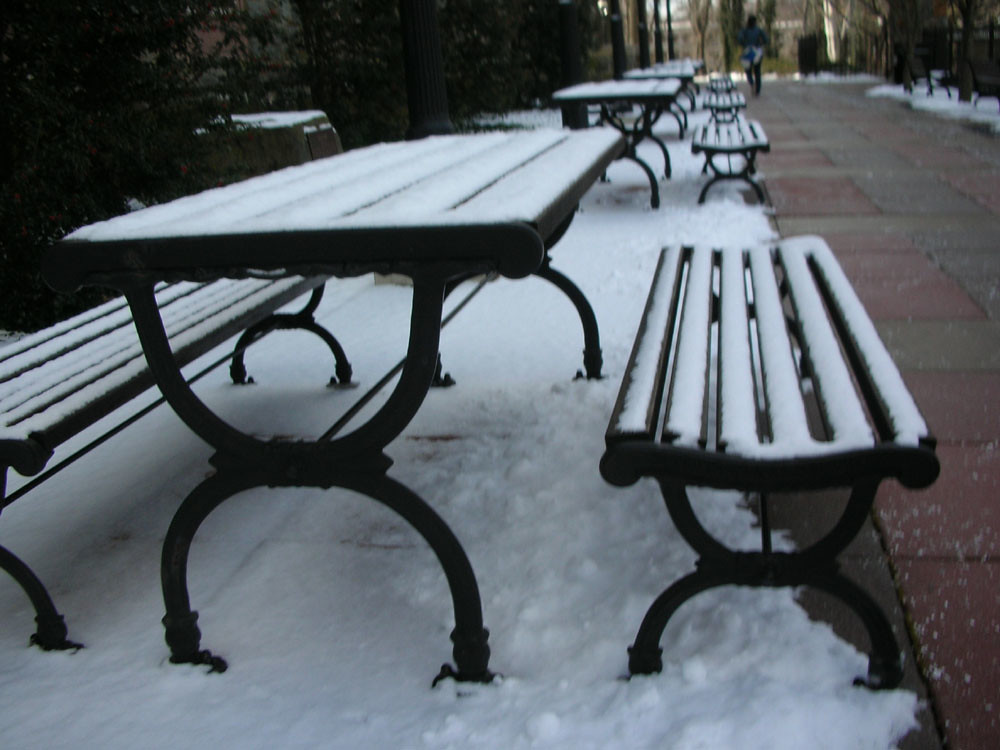This color photograph captures a snowy park scene featuring a series of black picnic tables and benches arranged in a row, extending into the background. Each table is accompanied by two matching benches on either side, all adorned with thin, slatted tops. The distinctive hourglass-shaped legs of the furniture give them a unique, elegant appearance. An inch-thick layer of fluffy, white snow covers the tables, benches, and ground beneath them, further emphasizing the serene, wintry atmosphere. To the right of the image, a stone pathway, paved with alternating red and grey square bricks, remains mostly clear except for a light dusting of snow. In the distance, a person dressed in black pants and what appears to be a sweatshirt tied around their waist can be seen walking along the path. The left side of the image is populated with trees, and in the upper left, there is a hint of a darker area with faint traces of snow. Additionally, the blurred horizon reveals a mix of more trees and possibly city buildings peeking through.